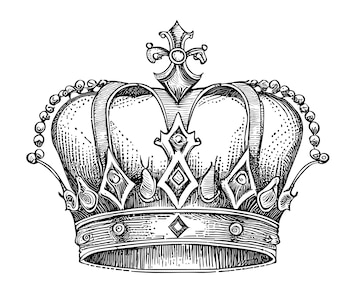The image is a detailed black and white pencil drawing of a luxurious crown, reminiscent of those worn by British royalty. The crown features an ornate floral cross at the top, flanked by pearls that cascade down the sides. Intricate floral patterns adorn the front of the crown, adding to its regal elegance. The base of the crown showcases a series of diamond shapes and circular patterns, which likely represent embedded jewels, with five prominent stones visible. The rim of the crown is decorated with a distinctive wood grain pattern, enhancing its intricate design. The interior of the crown appears to depict fabric, highlighting the exquisite craftsmanship of the piece.